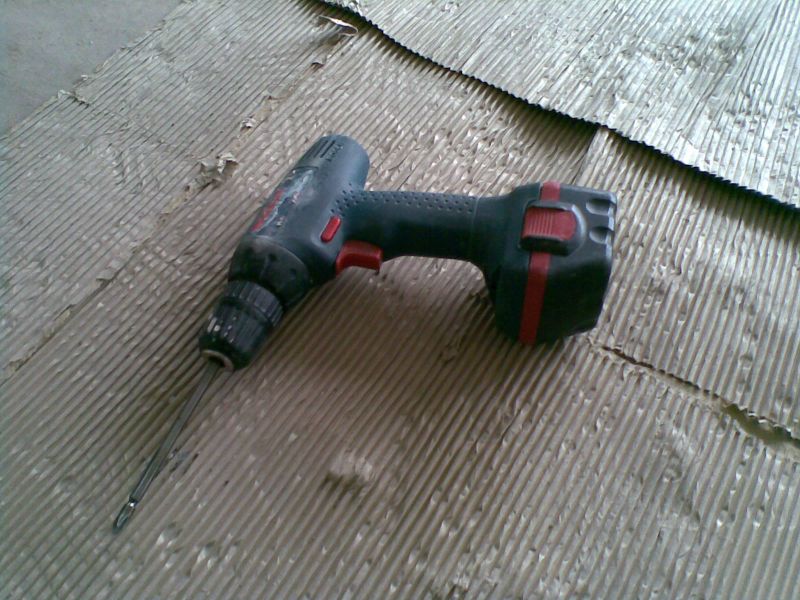This image showcases a cordless electric drill predominantly in black with red accents, such as a startup button and trim lines, lying on a piece of weathered, corrugated cardboard. The drill, which appears somewhat dirty, features a long Phillips head screw bit already attached. The cardboard itself is wrinkled and punctured, and it rests on a grey concrete floor partially visible in the upper left corner of the picture. The scene is brightly lit, with sunlight causing a noticeable glare in the upper right corner and casting reflections on the drill and the cardboard.